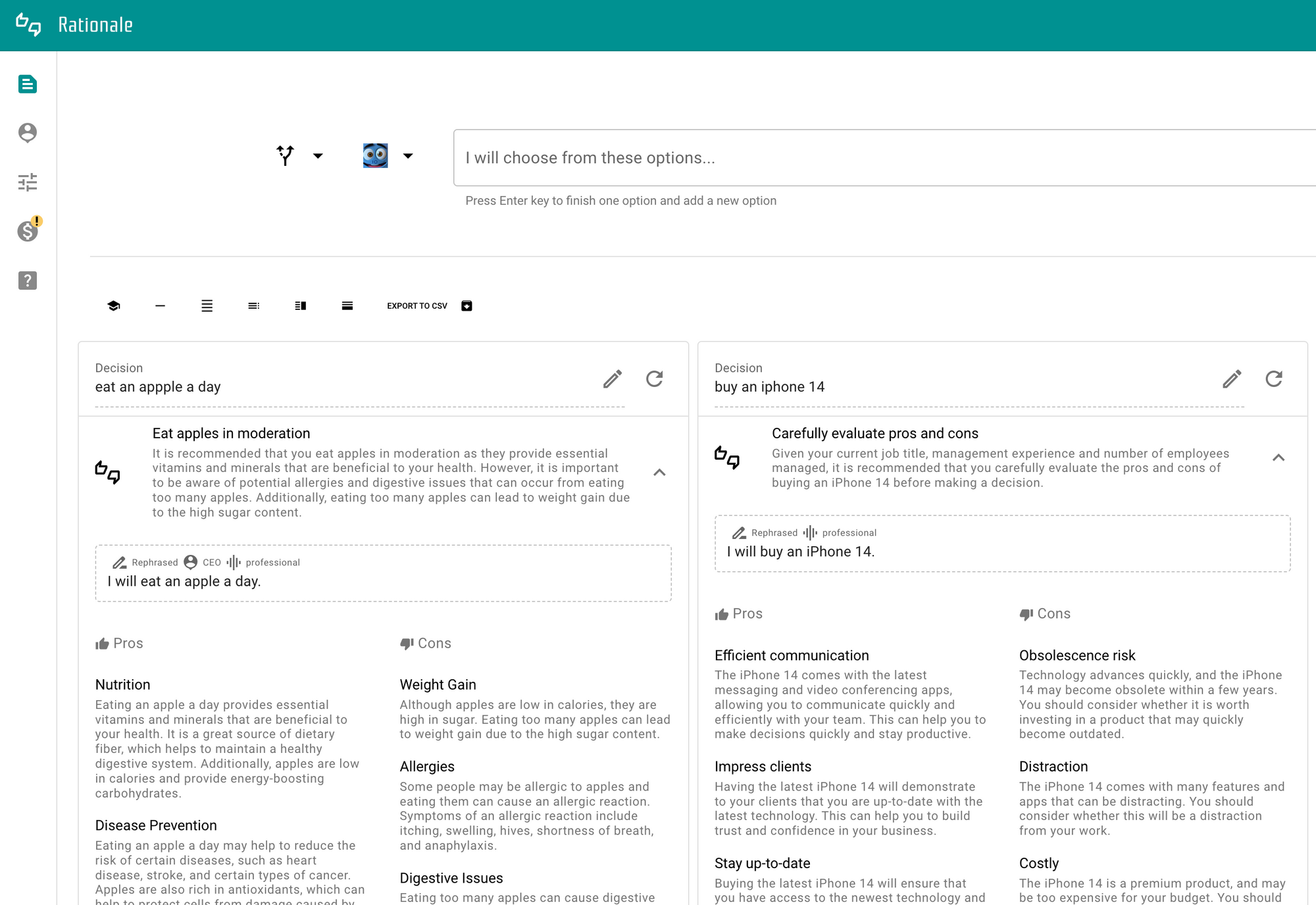This image depicts the settings section of a website template. The top of the page features a green navigation bar displaying the word "Rationale" in the upper left corner, along with a logo that includes thumbs up and thumbs down buttons in white. On the left sidebar, several icons are vertically arranged: a piece of paper, a user icon, a filter button, a dollar sign symbol, and a question mark within a box, which likely represents help or Frequently Asked Questions (FAQ).

Moving to the right side, the main content area has a white background. At the top of this section, there's a box with several icons aligned to its left, with the text "I will choose from these options" inside the box. Below this box, the page is divided into multiple sections containing black text with titles above them. Additionally, both columns have an "edit" button and a "refresh" button positioned at the top.